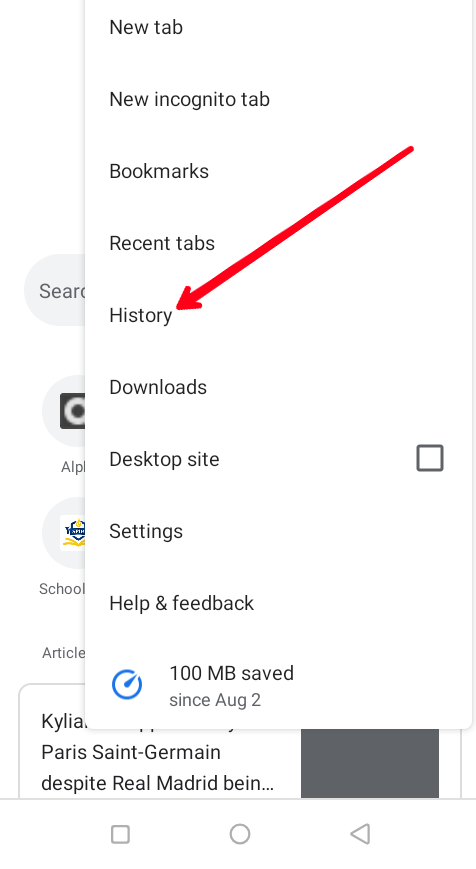This photograph captures a mobile phone screen displaying the browser menu of an open tab. The browser's menu lists several options in black font at the top, starting with "New tab," followed by "New incognito tab," "Bookmarks," "Recent tabs," and "History." A hand-drawn red arrow points towards the "History" option. The menu continues with "Downloads," "Desktop site"—next to which there is a clickable square indicator—"Settings," and "Help and feedback." At the bottom of the menu, a message indicates that the user has saved 100 MB of data since August 2nd. Partially visible behind the menu is the browser's default page, featuring a cut-off search bar at the top, various bookmarked apps and websites, and the beginning of a news headline: "Paris Saint-Germain despite Real Madrid," which is also partially cut off.